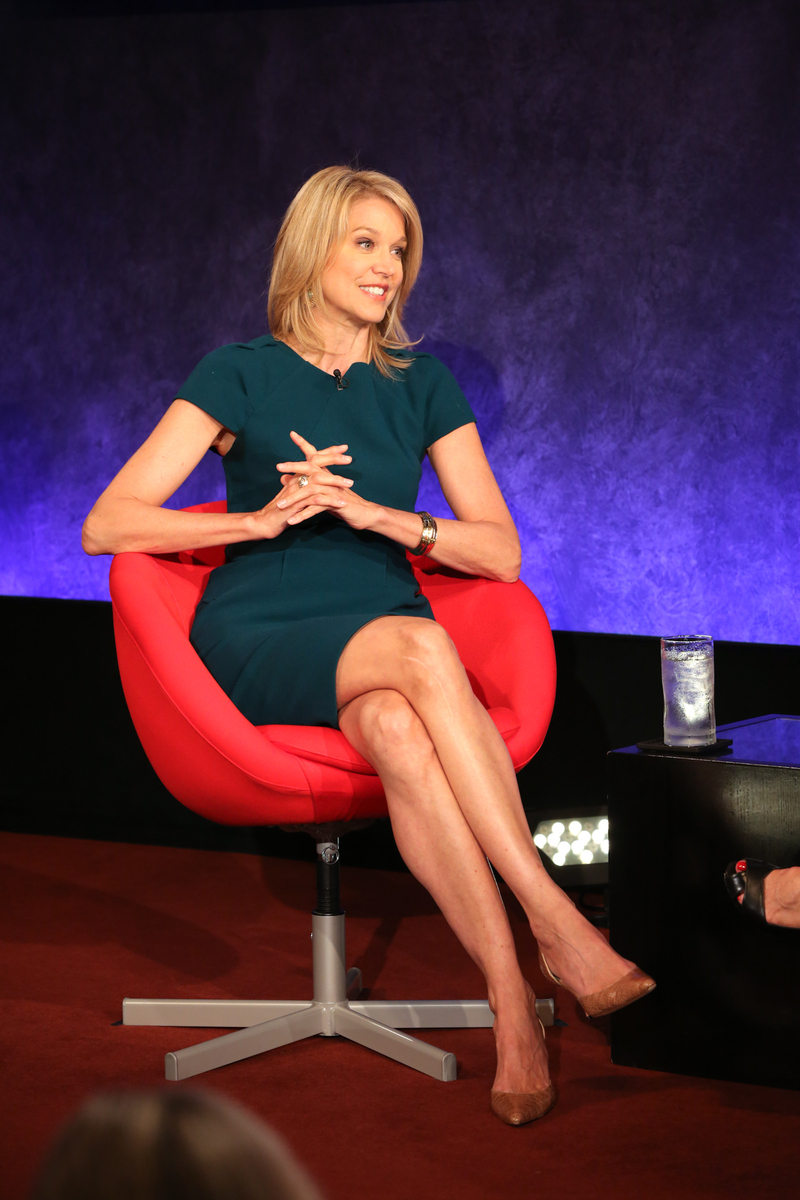The photograph captures a slender, blonde woman sitting in a rounded red chair featuring a single leg extending into a five-point base. The setting appears to be a studio with a blue background and red carpet. The woman, who seems to be either an interviewer or interviewee, is dressed fashionably in a short-sleeved green dress that falls to her calves. Adorning her left arm are silver or gold bangles, and on her right hand, she wears a prominent gold wedding ring. Attached to the collar of her dress is a small, knuckle-sized lapel microphone, pointing upwards. Her tan-colored high heels complement her attire, and she sits with her legs crossed, her hands lightly clasped on her lap. Smiling and looking off to the side as if conversing with someone, she appears engaged and attentive. Next to her is a small black square table holding a glass of ice water on a black coaster. In the periphery of the image, there is a glimpse of another woman's foot adorned with black heels and red toenail polish, hinting at an interview or discussion setting attended by more than one person.